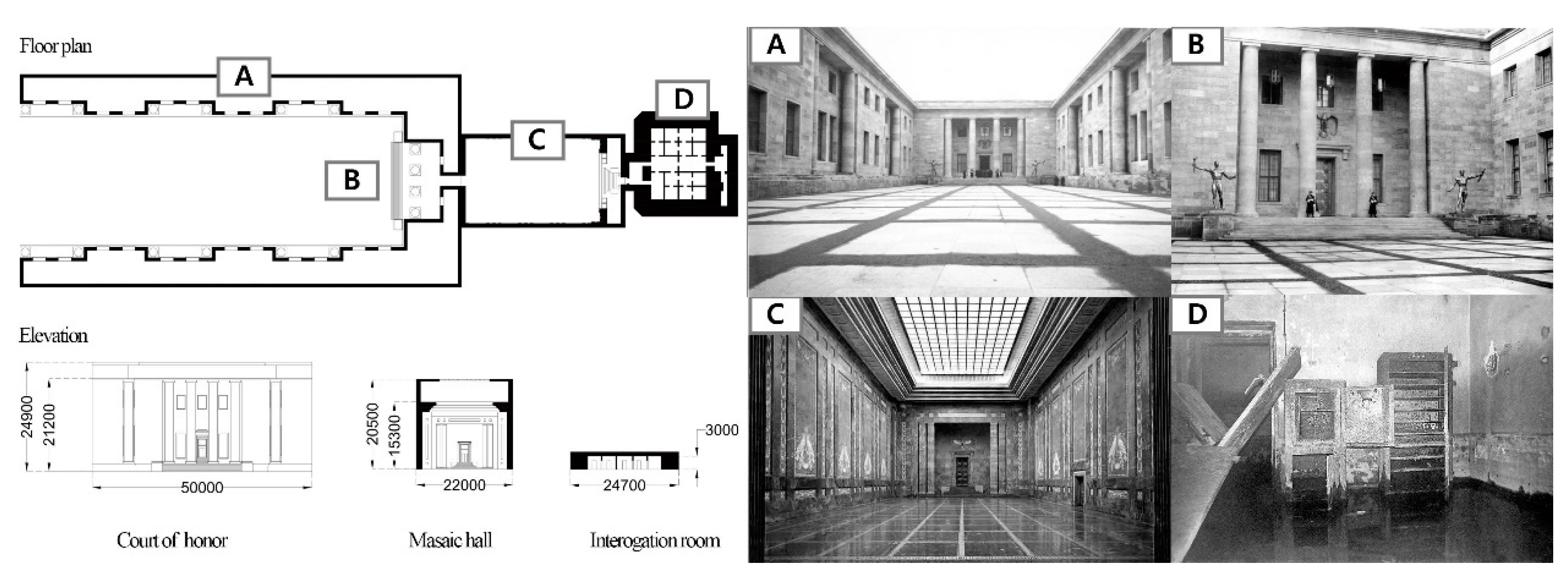The image is a detailed multi-part illustration, divided into two main sections: a blueprint on the left and four photographs on the right. In the upper left corner, titled "Floor Plan," there's a line drawing that showcases three rooms labeled A through D, connected by a long corridor. Beneath this floor plan, another diagram labeled "Elevation" provides a scaled view of these three rooms: the Court of Honor, the Messiah Call, and the Interrogation Room.

On the right side of the image are four black-and-white reference photos labeled A, B, C, and D. Photo A captures a courtyard view. Photo B shows the far end of that same courtyard, featuring three distinct columns. Photo C offers an interior view of the building observed in photo B, with detailed architectural features, while photo D displays the building that stands opposite to the one in photo C.

The elevation diagram highlights the grandeur of the Court of Honor with what appears to be significant lighting and spaciousness. Meanwhile, the Messiah Call and the Interrogation Room are also seen in the floor plan and elevation but presented with a contrasting focus— the Interrogation Room is more minimalist, featuring a small desk and cabinet, in stark contrast to the more elaborate Messiah Call. This overall collection of images effectively shows both the architectural plans and the corresponding real-life structures in meticulous detail.